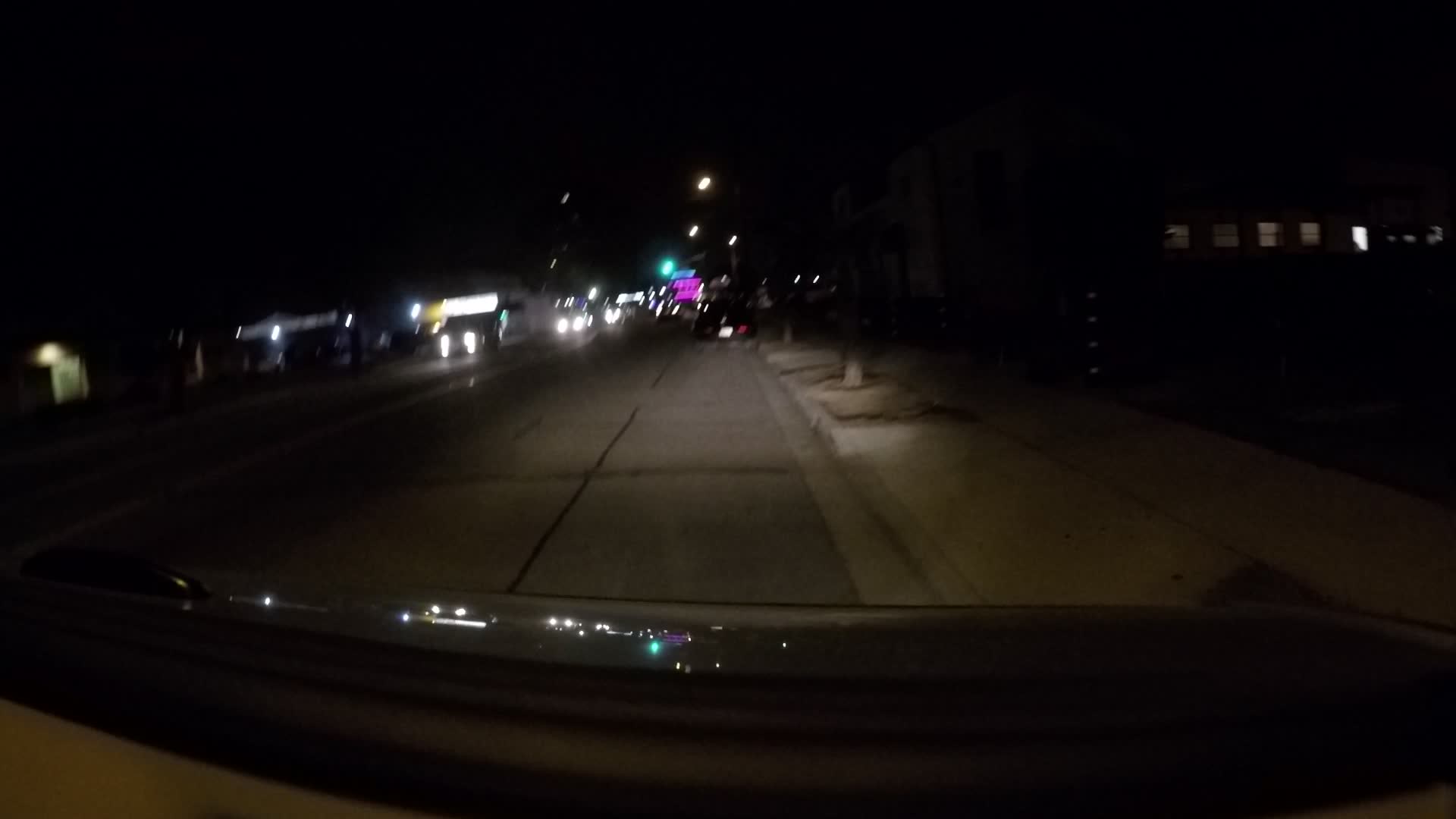In the dimly lit, blurred night photo taken from inside a car, likely through the windshield, a faint outline of the dark brown dashboard is visible. The scene outside reveals a black road stretching ahead under an equally dark sky. In the background, a myriad of lights illuminates the area, hinting at nearby stores, buildings, and street lamps. On the left, the headlights of oncoming vehicles suggest movement on a multi-lane road, potentially with a toll station overhead, as several illuminated lanes appear busy with cars. To the right, a sidewalk and curb are faintly discernible, leading off toward more lights in the far distance. A dark car is parked about 20 feet ahead on the right side, against the sidewalk. Additional elements include a dirt patch lining the street with planted trees, large street lamps, and a prominent purple sign possibly for traffic direction. The general surroundings indicate a commercial area rather than residential.